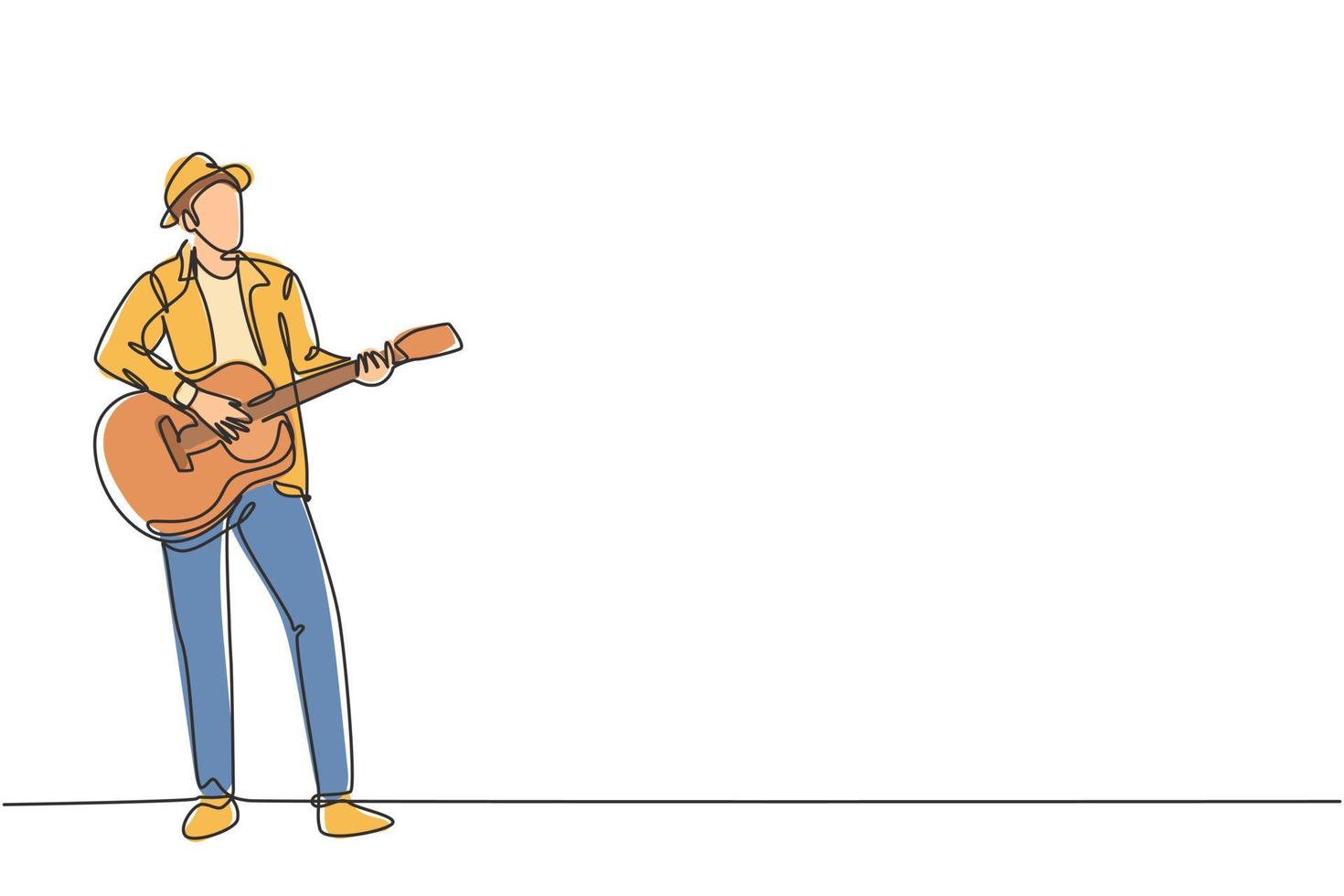The image features a simple line art drawing of a male figure positioned towards the left side of a predominantly white background, with a straight black horizontal line at the bottom representing the ground. The man, who lacks any facial features, has short brown hair peeking out from under a mustard yellow hat with a brim. He is dressed in a long-sleeved mustard yellow jacket over a lighter yellow shirt, blue jeans, and mustard yellow shoes. He is standing upright playing a guitar, which is light brown with a slightly reddish hue near the strings. One hand of the figure is on the neck of the guitar while the other is positioned on the body of the guitar.